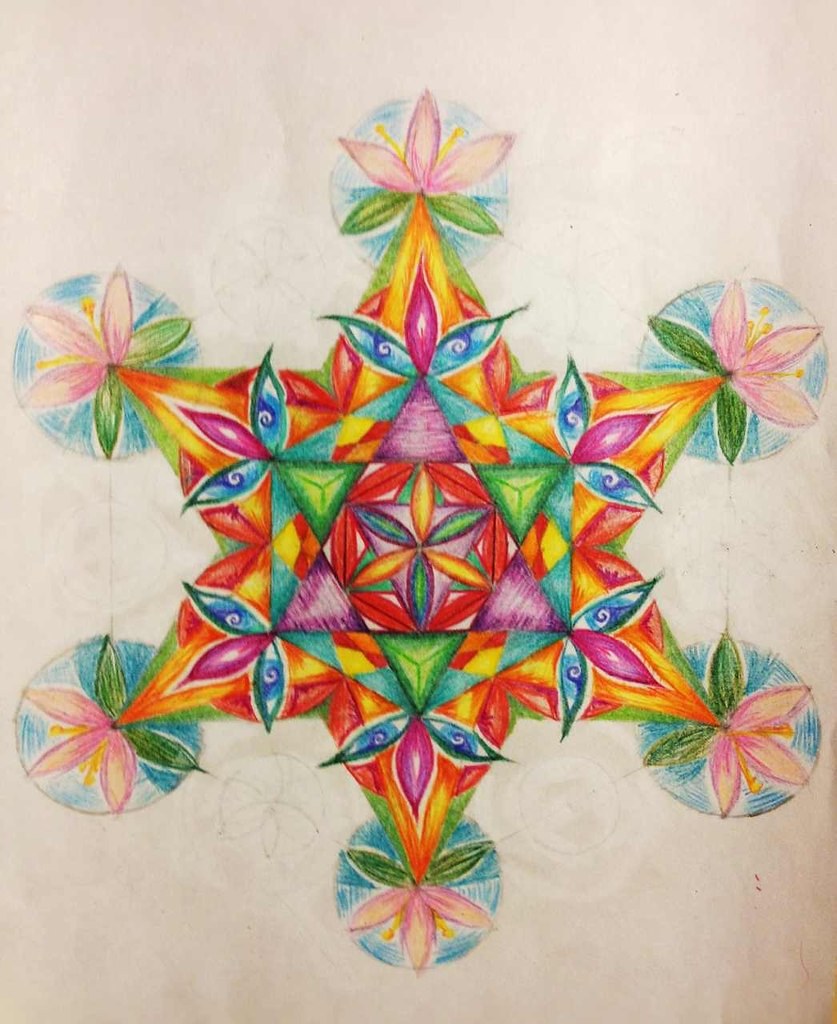**Detailed Description of the Image Drawing:**

The image features a top-down, bird's-eye view of a drawing on a white piece of paper. The drawing is meticulously coloured, with pencil line outlines enhancing its intricate design. The colourful artwork boasts a rich palette, including hues of green, orange, red, yellow, purple, pink, cyan, light blue, dark blue, light pink, and more.

At the heart of the drawing is a striking six-pointed star. Each point of the star is adorned with a bluish circle, from which emerge five petals. The three upper petals are rendered in shades of pink, while the two lower petals are depicted in a deeper green.

This central star is segmented into various colourful patterns. Starting from the tips of the star points, the sequence of colours transitions from green to orange, yellow to red, continuing with blue, orange, red, yellow, and green. This radiating pattern leads to the very centre, a red hexagon.

Inside this central red hexagon lies an additional star shape, composed of six petals arranged in a harmonious star formation. This star is set within a triangle shaded in blue and purple, which overlaps and contrasts with a green triangle. The blue triangle is oriented with its tip facing downward, while the green triangle's tip points upward.

The entire design showcases a very ornate and intricate pattern, reflecting a high level of detail and an exquisite balance of colours.